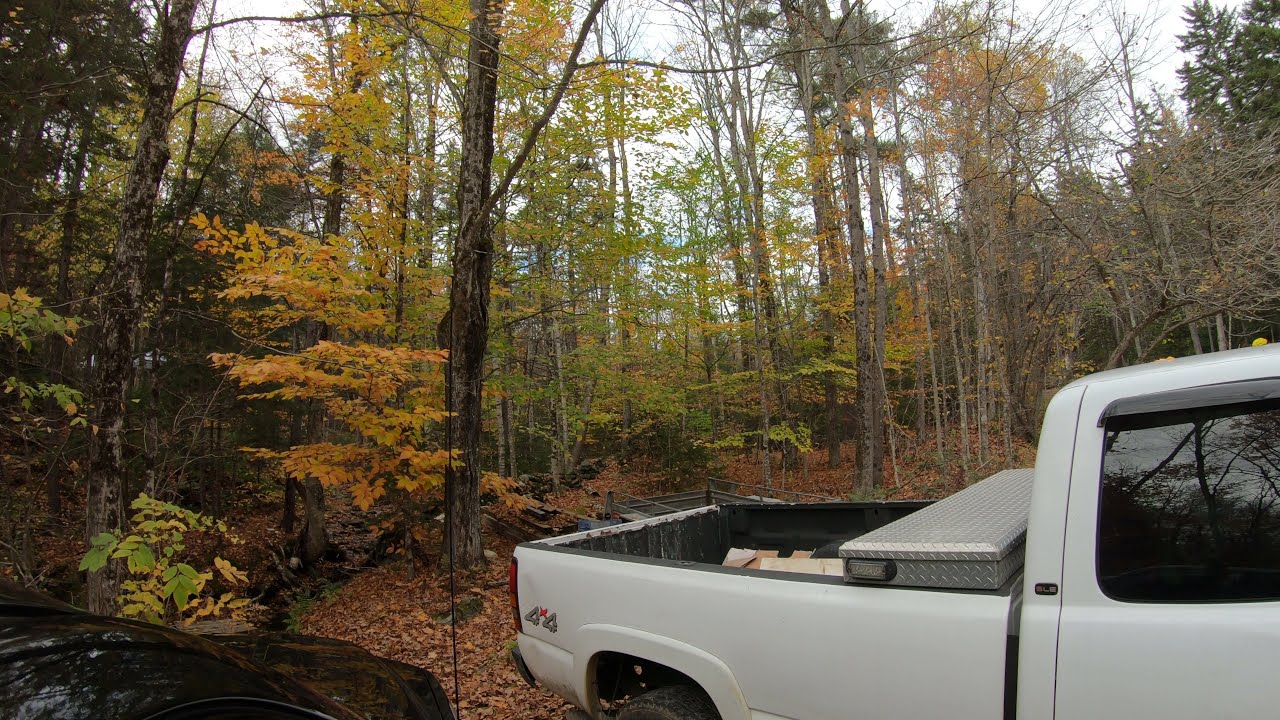In this photograph, a white 4x4 pickup truck is prominently positioned in the bottom right corner of a picturesque autumn forest. The truck's bed is filled with wooden logs and features a diamond-plated tool chest. Next to it, partially visible in the bottom left corner, is a black vehicle, adding an element of mystery to the scene. The forest is alive with an array of colors, showcasing trees with leaves that are various shades of yellow, green, red, and golden, along with some bare branches indicative of fall. The ground is carpeted with a thick layer of fallen leaves, further emphasizing the season. Scattered around the forest floor are additional wood pieces and what appears to be construction equipment, hinting at recent activities. The sky above is a bright white, partly cloudy, illuminating the scene with soft, diffused daylight.